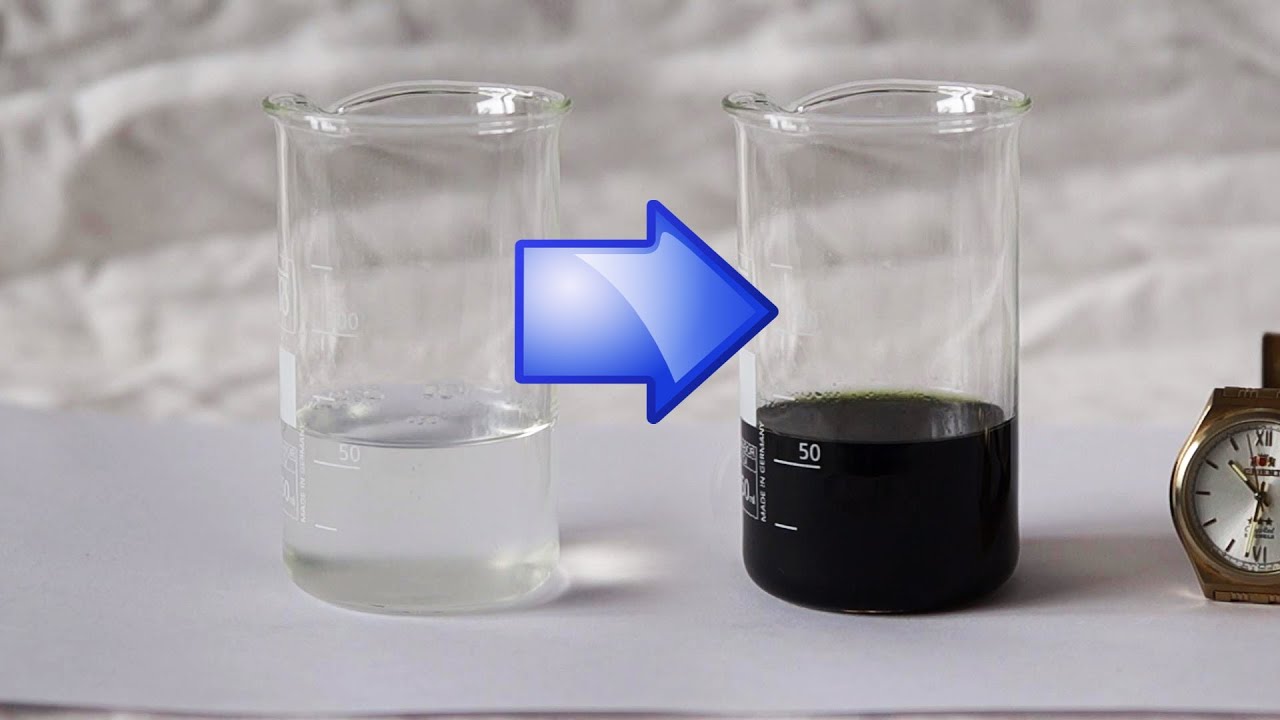This detailed photograph, possibly from a scientific journal, features two labeled milliliter glass beakers situated on a table, both showing signs of condensation. The beaker on the left contains a clear liquid resembling water, while the beaker on the right holds an ominously black liquid that could be motor oil or dye. Superimposed over the image, a stylized blue arrow, designed with a gradient from dark blue edging to a lighter blue point, directs attention from the left beaker to the right one, possibly indicating that the contents of the left beaker are to be poured into the right. To the right of the dark liquid beaker lies a watch, displayed against a slightly out-of-focus background that appears to be a sheet or mattress. The watch shows a time of 10:33, with the second hand nearing midnight.